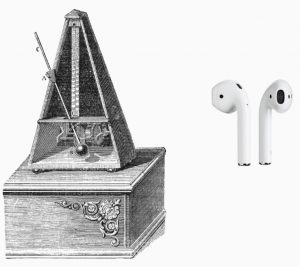The image consists of two distinct parts set against a light gray or very light blue background. On the left side, there is a detailed black and white line drawing of an old-fashioned metronome. The metronome features a large, cuboidal base adorned with some designs, supporting a triangular top that has a vertical striped metal piece running down its center. A pointer or bar, which swings to indicate the tempo, is currently pointing to the top left. On the right side, the image showcases a pair of white earbuds, each with small black sound holes and a silver end piece. One earbud is oriented with its rounded part facing left, while the other faces right.